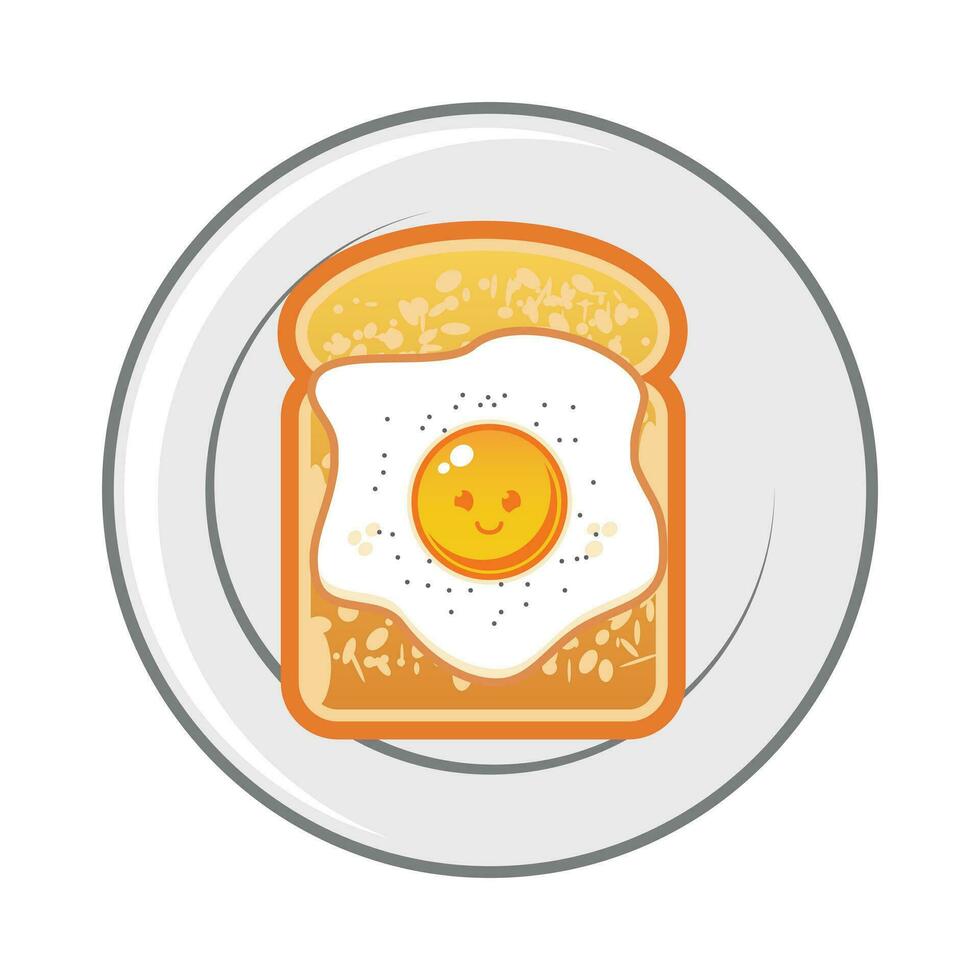The image is a cartoon-style drawing that shows a top-down view of a gray plate with a light gray inner circle. On this plate sits a piece of toast, outlined in orange with a tan to brown gradient and some yellowish-orange spots indicating toasting or butter. Atop the toast lies a sunny side up egg, outlined in orange, with pure white egg whites sprinkled with black pepper specks. The golden-yellow yolk features a smiling face with two white dots on the upper left and a subtle orange crescent on the right, giving it an emoticon-like expression. The overall art is modern and reminiscent of digital animation or AI-generated clipart, utilizing a minimalistic yet colorful palette primarily in shades of gray, yellow, black, white, and orange.